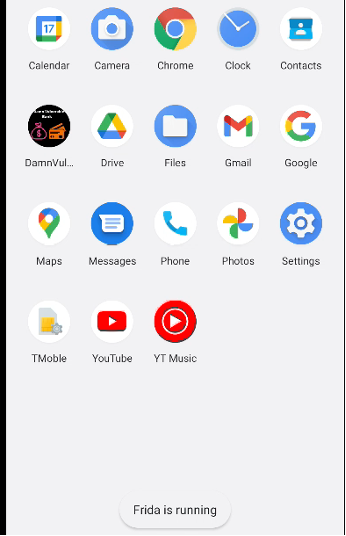The image depicts a smartphone screen, featuring a neatly arranged list of applications. Judging by the icons, it appears to be a device running either a Google or iPhone operating system. The background is a subtle light gray or white, setting a clean and minimalistic tone.

At the top of the screen, the Calendar app icon is prominent, showcasing the number 17 within a rainbow-colored square. Adjacent to it is the Camera app, represented by a classic camera icon. Other notable applications include Google Chrome, Clock, and Contacts. 

Interestingly, the display includes "Danville Drive," likely a localized naming variation for Google Drive, alongside standard apps like Files, Gmail, Google, Maps, Messages, Phone, Photos, Settings, T-Mobile (stylized without the "I"), YouTube, and YouTube Music (abbreviated as UT Music with its distinctive circular logo).

The icons are systematically arranged into four rows, each containing five apps, except for the last row, which holds only three. At the bottom of the screen, there is a small text bubble indicating "Frida is running." This detail might suggest some background activity or notification specific to the phone's user.